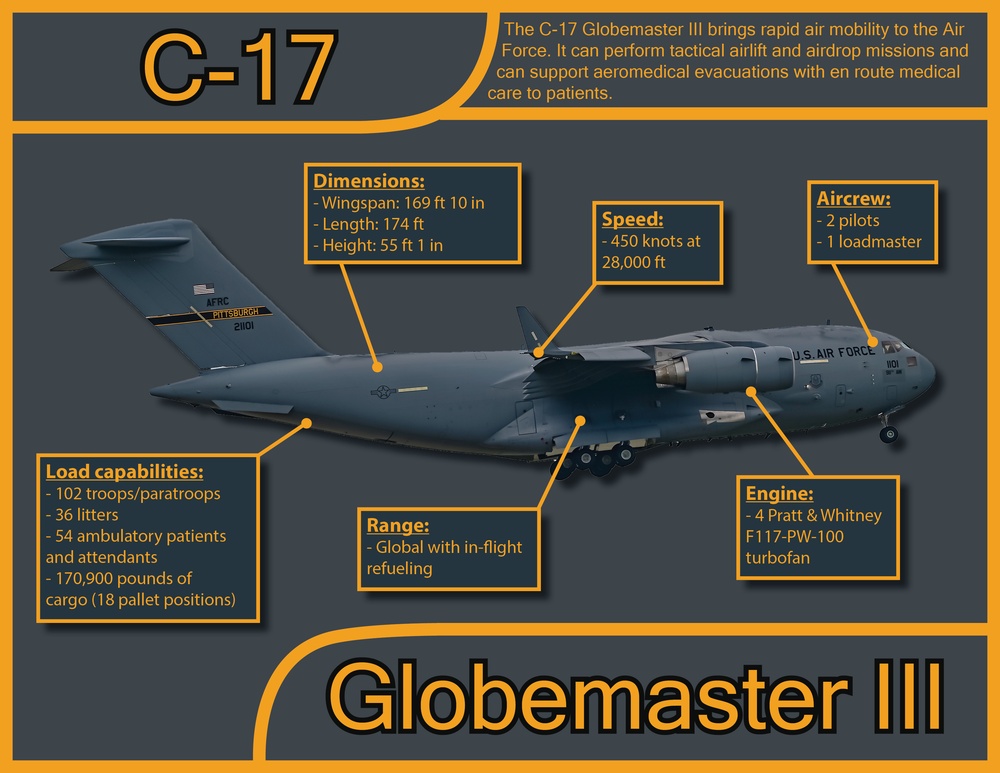The image is a detailed color illustration of a C-17 Globemaster III jet, prominently centered and facing to the right. Titled "C-17" with the subtitle "The C-17 Globemaster III brings rapid air mobility to the Air Force," this diagram highlights the aircraft's multifunctional capabilities, including tactical airlift, airdrop missions, and aeromedical evacuations with en-route medical care. The dark gray jet, marked with the text "U.S. Air Force" near the cockpit, is surrounded by blowout boxes labeling various parts and specifications: the aircrew (two pilots and one loadmaster), speed (450 knots at 28,000 feet), dimensions (wingspan of 69 feet, 10 inches; length of 174 feet; and height of 55 feet, 1 inch), load capabilities (102 troops or paratroops, 36 litters, 54 ambulatory patients and attendants, or 170,900 lbs of cargo), range (global with in-flight refueling), and engine type (F117-PW-100 Pratt & Whitney turbofan). The image further emphasizes its illustrative style combined with graphic design by framing the content within a gold border and using bold gold text for key labels, including "GLOBEMASTER III" at the bottom right. The background features a light gray gradient, enhancing the visual clarity and professional presentation of the aircraft's details.